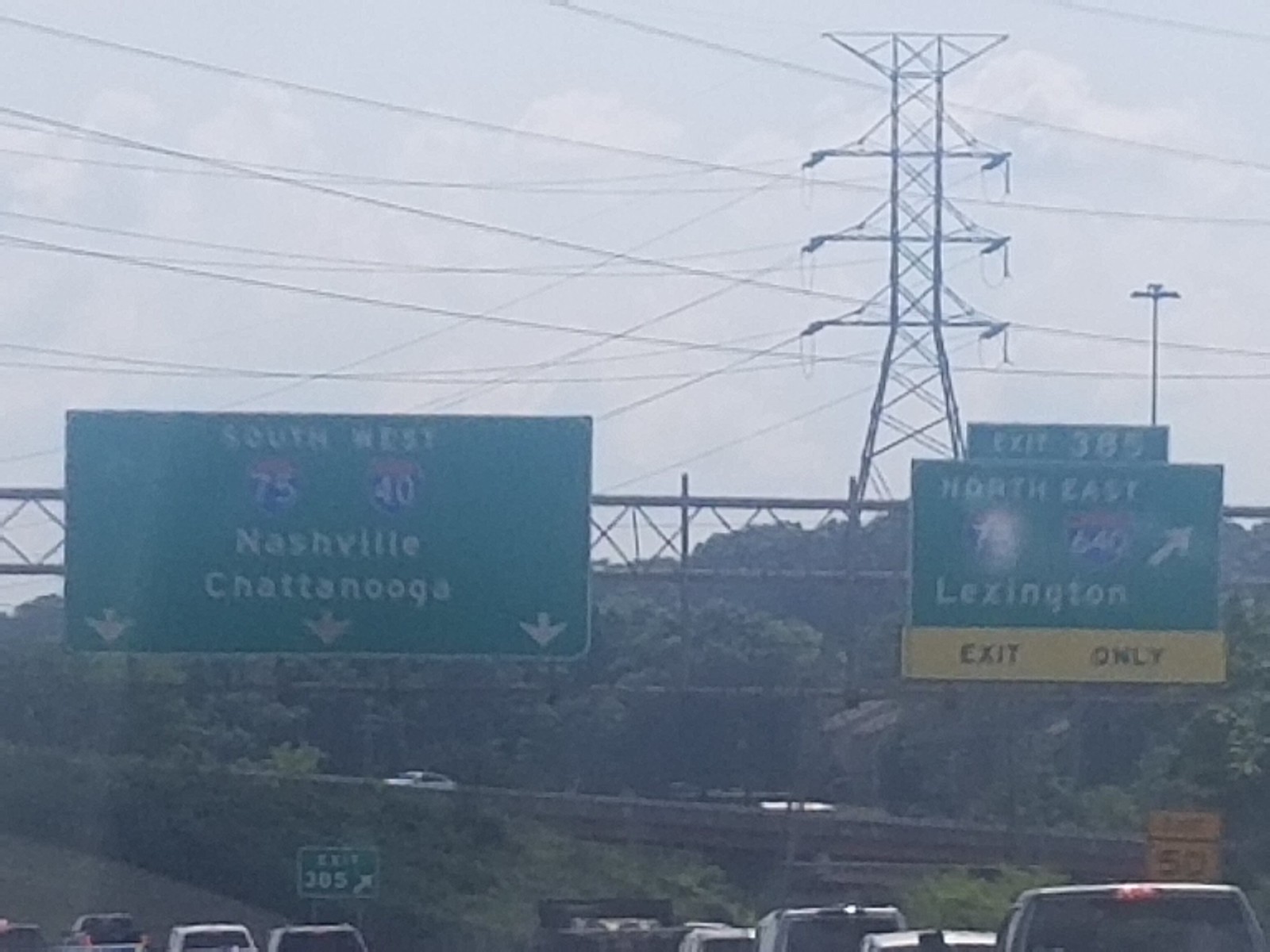This photograph captures a busy highway scene under a light gray, slightly cloudy sky. In the center of the image are two prominent green highway signs mounted on large, silver arms that stretch across multiple lanes of traffic. The left sign directs drivers to "South 75/West 40" toward "Nashville" and "Chattanooga," featuring the iconic blue-and-red interstate shields. Below these names are three white arrows pointing down, indicating the correct lanes. On the right side, a sign indicates "Exit 385 Northeast 75/640" toward "Lexington," with a white arrow pointing up and to the right, and a yellow "Exit Only" rectangle at the bottom. In the background, there's a massive electrical tower with numerous wires crisscrossing the scene. Traffic fills the highway, including a variety of cars and trucks, and an additional small green sign for "Exit 305" is visible amid the congestion.